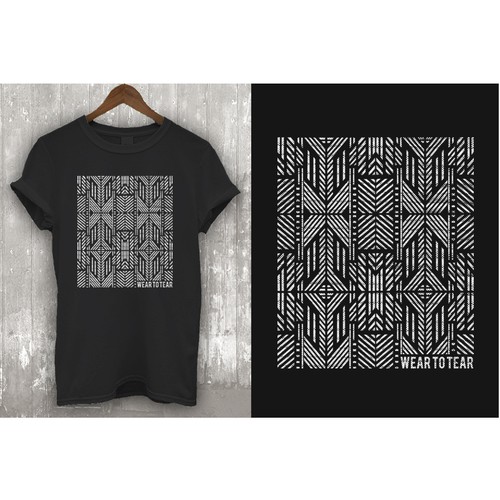The image is composed of two sections side-by-side. On the left, there is a black t-shirt with rolled-up sleeves hanging on a wooden hanger, partially visible against a rustic white and gray wooden wall. The t-shirt features a perfectly square graphic in the center, showcasing an intricate black and white geometric design. This design includes various shapes such as diamonds, Xs, triangles, and arrows, all arranged in zigzag and diagonal patterns. On the right side of the image, a zoomed-in view of the square graphic is presented against a black background. The close-up reveals the detailed geometric patterns more clearly, and small white text at the bottom right corner of the design reads "where to tear."